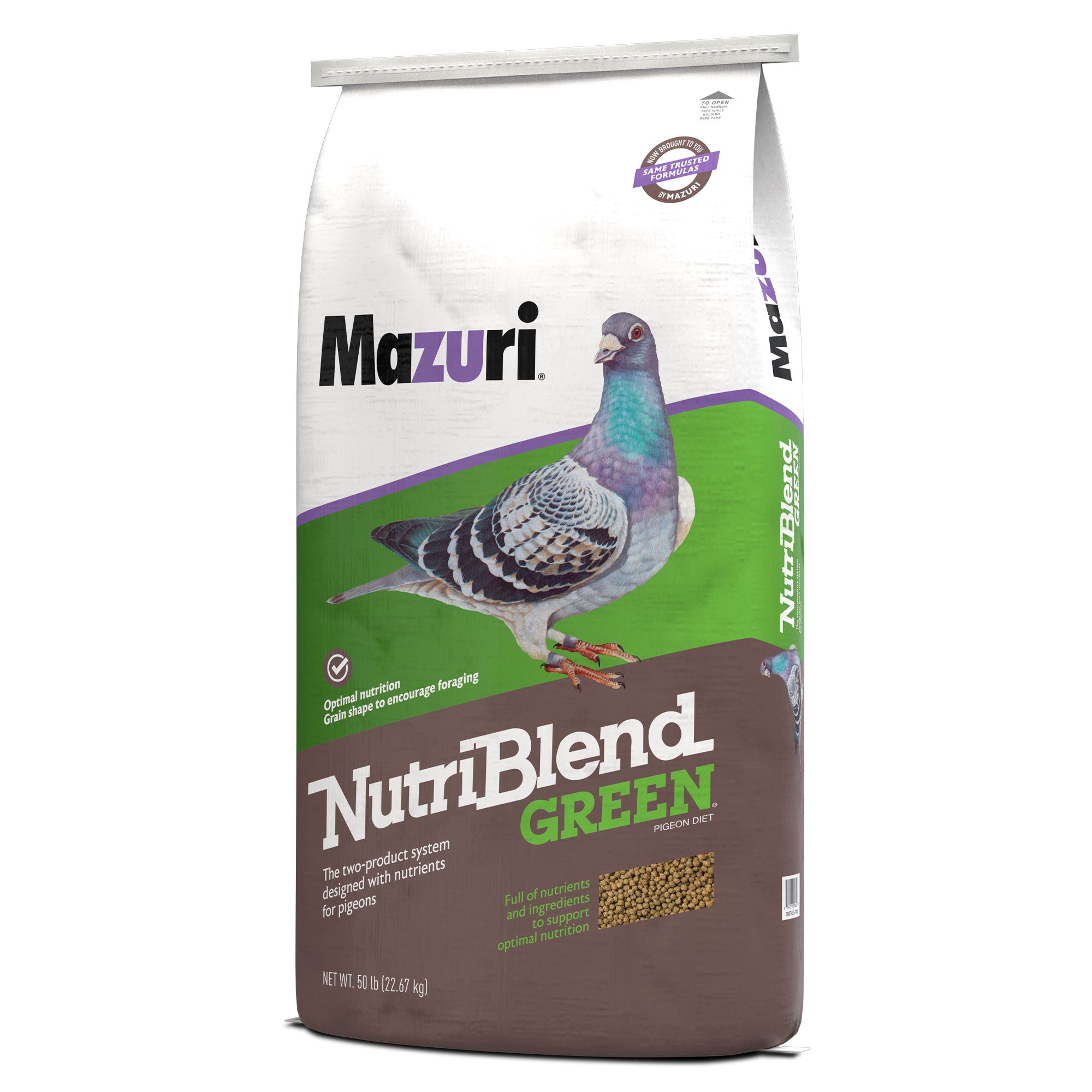The image depicts a vertically oriented, 50-pound sack of birdseed designed for pigeons, branded by Mazuri. The bag features a three-color design: white at the top with a purple stripe at an angle, followed by green, and concluding with a brown band at the bottom. In the middle, there is an image of a pigeon with green chest and tail feathers. The product is identified as "Nutriblend Green Pigeon Diet," highlighted beneath the pigeon illustration. A unique feature of the packaging is a small transparent window near the bottom that reveals the birdseed's pellet form. The bag includes a string closure at the top, allowing easy opening by pulling the string. The packaging emphasizes that this pigeon feed is formulated with optimal nutrients to support pigeon health.